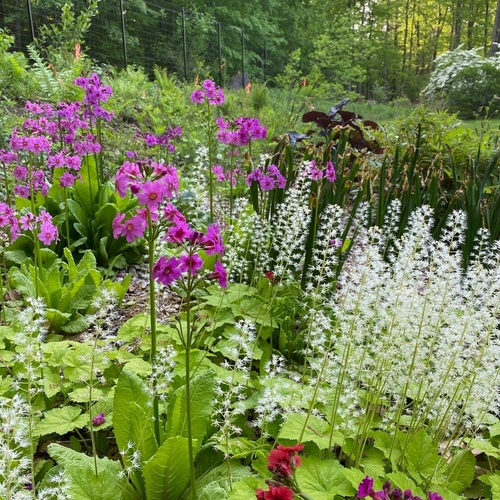This captivating outdoor photograph showcases the enchanting beauty of an overgrown forest. Towering, dense green trees dominate the background, creating a lush canopy that hints at the forest's depth and richness. A rustic wooden fence lines the edge of the forest, partially concealed by the riotous growth of the surrounding vegetation. In the foreground, a vibrant meadow of wildflowers bursts into vivid colors, featuring delicate pink, pristine white, and deep blue blossoms. The scene exudes a sense of untamed wilderness, with the ground teeming with verdant life and a wild, exuberant feel. The overall image is a lively tapestry of green hues, evoking a profound connection to nature's raw, unmanicured splendor.